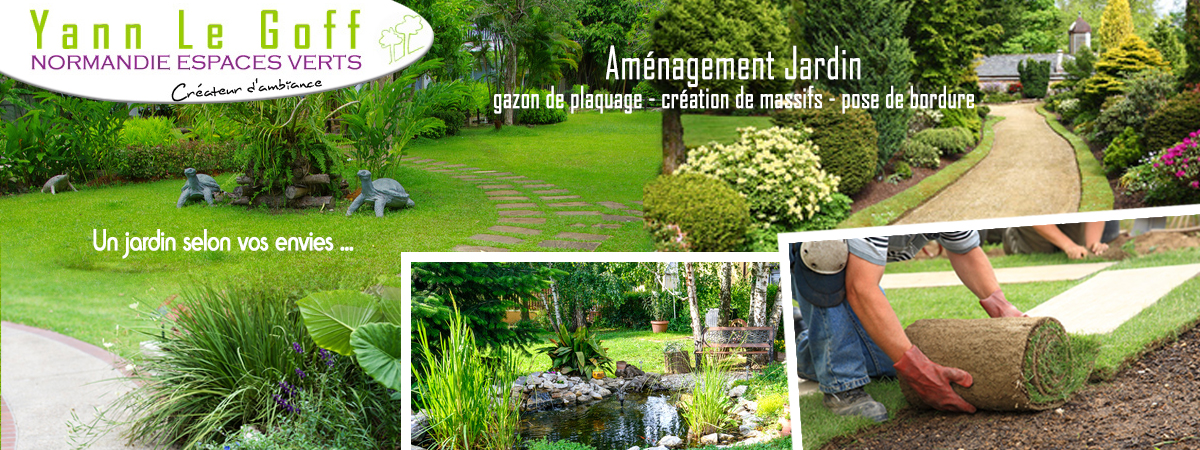The image depicts a meticulously landscaped garden scene, likely an advertisement for a landscaping business, prominently featuring the name "Yann Le Goff." The main photograph showcases a verdant, well-maintained yard with vibrant, bright green grass and a stone walkway leading through the space. The surrounding vegetation includes lush, trimmed shrubbery, purple flowers, and other greenery, indicating a high level of professional care. 

In the forefront, a man is unrolling fresh sod beside a stone path, suggesting active yard improvement. In the background, there's a pond framed by tall green plants and white stones, with a bench and a distinct white tree lined with brown bark nearby. Additional smaller images nestled in the bottom right of the main picture illustrate more detailed scenes from the garden. The text contains multiple references in French, such as "Normandy Espace Verts," "Un Jardin Sillon Vos Envies," and "Gazon des Locages," highlighting various landscaping services including turf installation, garden creation, and border design. 

The scattered yet harmonious placement of objects and plants create a visually appealing and well-organized outdoor space, emphasizing the expertise and comprehensive service range of the landscaping business.